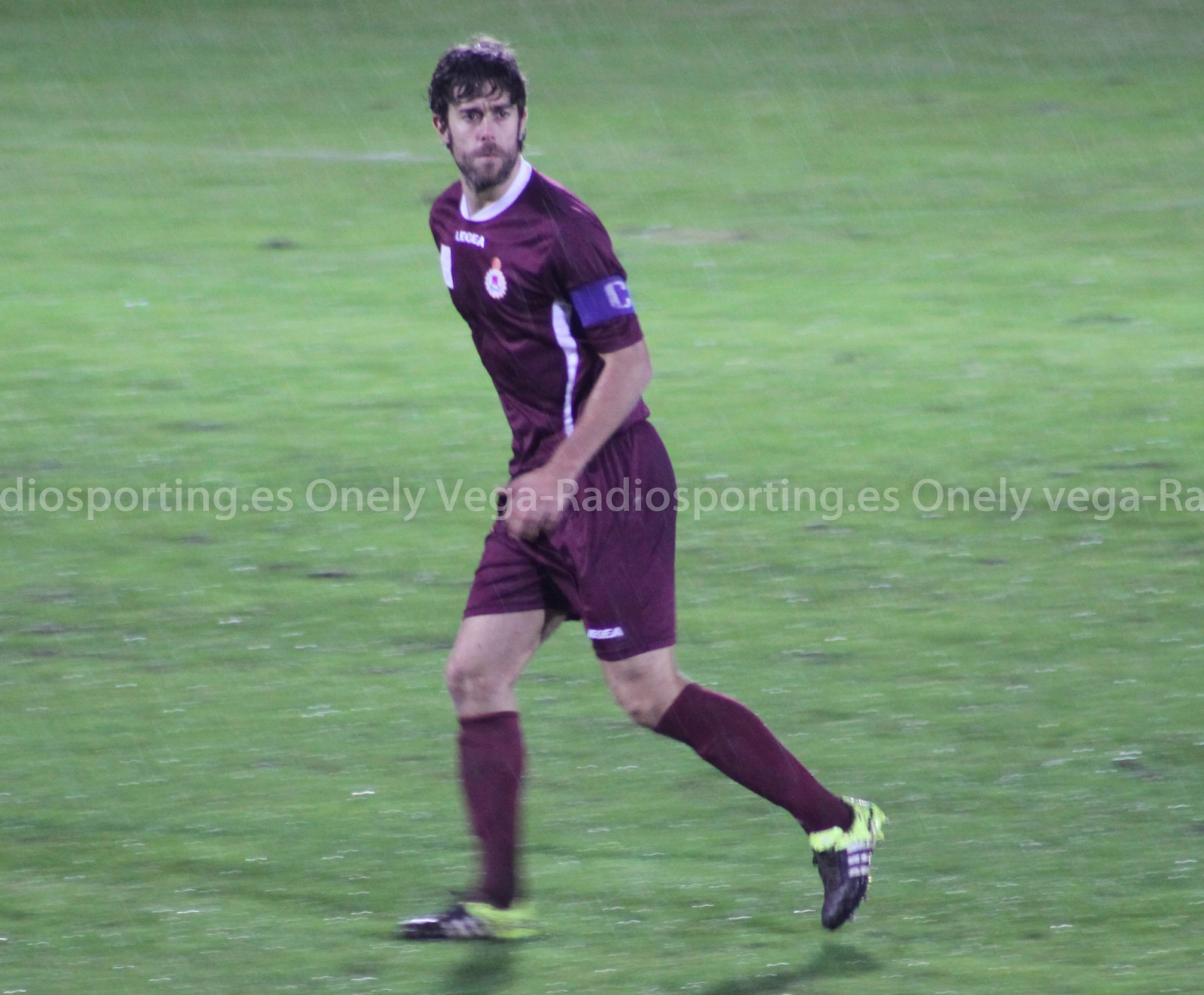The photograph captures a young soccer player, a white male with dark, damp hair, suggesting he's either been sweating or playing in the rain, as raindrops are visible in the image. He wears a dark burgundy soccer uniform with matching shorts and socks that reach up to his knees. A blue patch adorns his left arm. His cleats are distinctively bright with a fluorescent yellow back, black front, and three white stripes. The player is running across a lush green field, looking intently to his left with a serious expression on his face. Text repeating "onelevega-radiosporting.es" is visible in the background.